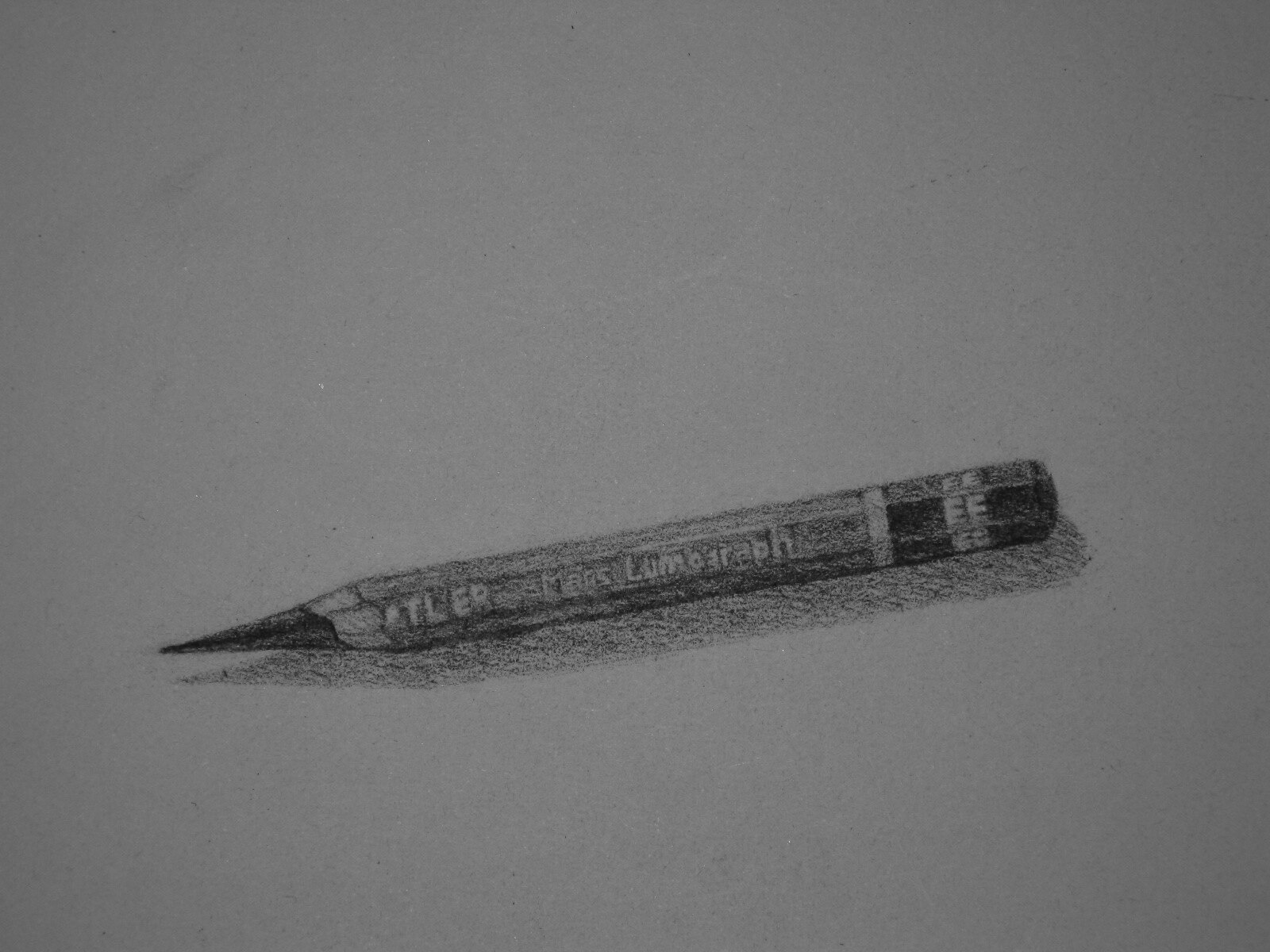This detailed sketch depicts a well-used pencil resting on a slightly dark grayish-white piece of paper. The pencil, sharpened to a precise point, appears to be about half its original length, suggesting extensive use. It is positioned diagonally, with the point slanting down to the left and the eraser end slanting up to the right. A shadow beneath the pencil indicates it is lying on a surface. The pencil bears the word "ATLER" in white, followed by "MANS" and "LUMOGRAPH." The stub or eraser end of the pencil is black, adorned with the repeating letters "E-E." The intricate details and thoughtful placement of the shadowing enrich the realism of the sketch.